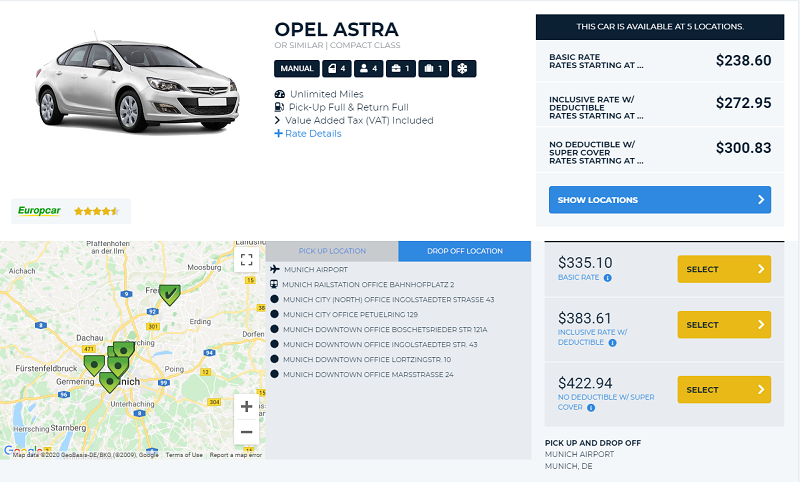The image features an Opel Astra, a popular rental car option in Europe. Various rental packages are at play here:

1. **Basic Rate**:
   - Cost: $238.60
   - Included Services: Unlimited mileage, pick-up full and return full fuel policy, value-added tax.

2. **Inclusive Rate**:
   - Cost: $272.95
   - Additional Coverage: Deductible rates included.

3. **Super Cover (No Deductible)**:
   - Cost: $300.83
   - Superior coverage with no deductible.

**Car Details**:
- Type: Four-door sedan
- Capacity: Four passengers
- Luggage: Space for two bags
- Season: Suitable for winter driving
 
The image specifies pickup and drop-off locations: Munich Airport for both, with rental pick-up policies emphasizing full tank returns. Alternative pricing is also indicated, listing a basic rate at $335, an inclusive rate at $383, and a no deductible package for $422.